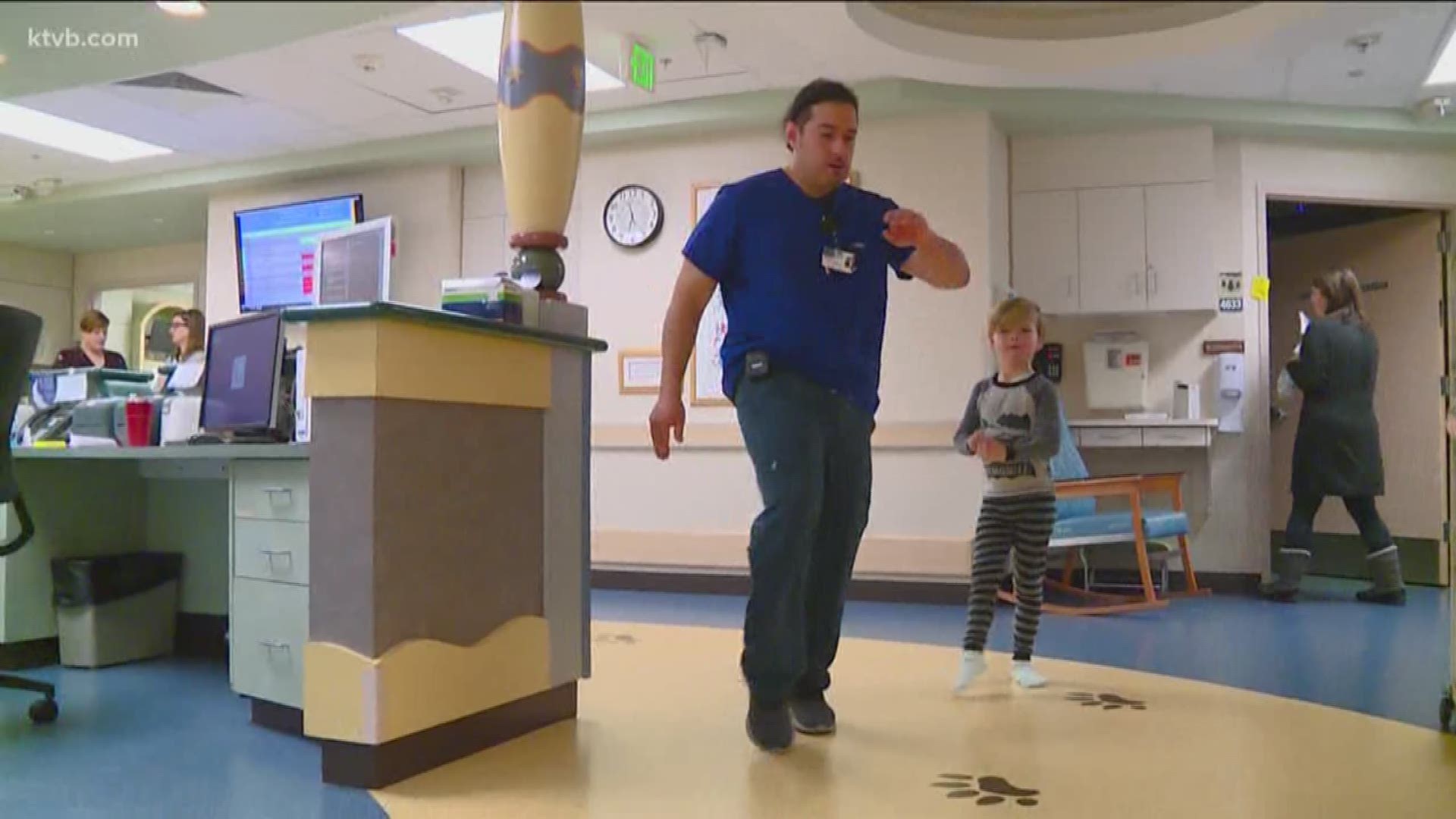In this detailed indoor scene, which seems to depict a hospital or clinic, a Caucasian man with short brown hair is seen walking through a corridor. He is dressed in a bright blue short-sleeve shirt and gray pants, with a lanyard bearing a white card hanging around his neck. Attached to his belt on the left side is a clicker, and his head is tilted slightly downward. His right arm is raised almost to shoulder level, with his hand in front of his chest, while his left arm hangs loosely by his side. Accompanying the man is a young child with blonde hair, around elbow height to the man. The child wears a gray pajama top with darker gray sleeves and matching gray and black striped bottoms, along with white socks—one foot flat on the floor and the other with the toe pointed down.

The floor in front of the man features painted paw prints, suggesting a child-friendly environment possibly in a pediatric section of the hospital. Behind the man and to his right, a young boy seems to be watching him, and on the far right of the image, a woman in a gray long coat and gray mucklucks with a white ring at the top is seen walking through a doorway. 

To the left, part of a nurse’s or administrative station is visible with a desk, computer, filing drawers, and a trash can underneath. An analog clock is mounted on the wall, and further left, a screen with blue and light green lines is visible, adding to the clinical ambiance. Above at the top, “ktvb.com” is superimposed in light text, hinting that this might be a still from a video.